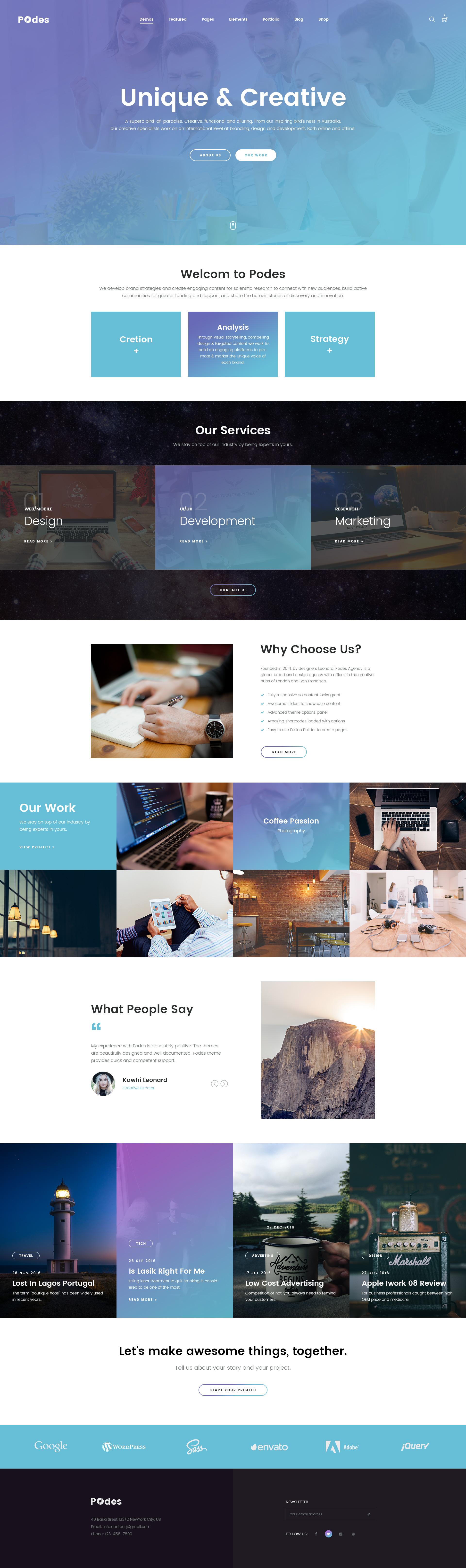**Screenshot of a Vibrant and Dynamic Website Homepage**

The homepage screenshot features a lively and engaging photograph of five people at the top, capturing a moment of joy and collaboration. A man and a woman are seated at a table, surrounded by three standing individuals. All five are laughing and cheering, focused on a white laptop in front of them. 

In the top left corner of the screen, the PODES logo appears in white text. The logo consists of a capital "P" followed by an "O" stylized to resemble a cracked CD, then lowercase letters "DES." 
To the right of the logo lies a navigation menu, also in white text, featuring the following options: DEMOS (underlined thinly in white), FEATURED, PAGES, ELEMENTS, PORTFOLIO, BLOG, and SHOP. 
In the top right corner are two icons: a white magnifying glass and a white shopping cart with a white numeral "2" above it, indicating two items in the cart.

The photograph beneath the header has a vibrant color overlay transitioning from purple in the top left to bright blue in the bottom right, forming a gradient at the center. 
Centered on the photograph is prominent white text that reads "UNIQUE & CREATIVE." Below this are two lines of thin white text: 
- "SUPERB BIRD/DASH OF PARADISE, CREATIVE, FUNCTIONAL, AND ALLURING."
- "From our inspiring bird's nest in Australia, our creative specialists work on an international level at branding, design, and development, both online and offline."

Beneath this text are two buttons:
- On the left, a translucent button with a thin white outline containing white text that reads "ABOUT US."
- On the right, a solid white button with blue text that says "OUR WORK."

At the bottom center of the photograph, a white mouse icon suggests further scrolling. Below this main image, the website layout continues, alternating between colored backgrounds and sections with photographs and text.